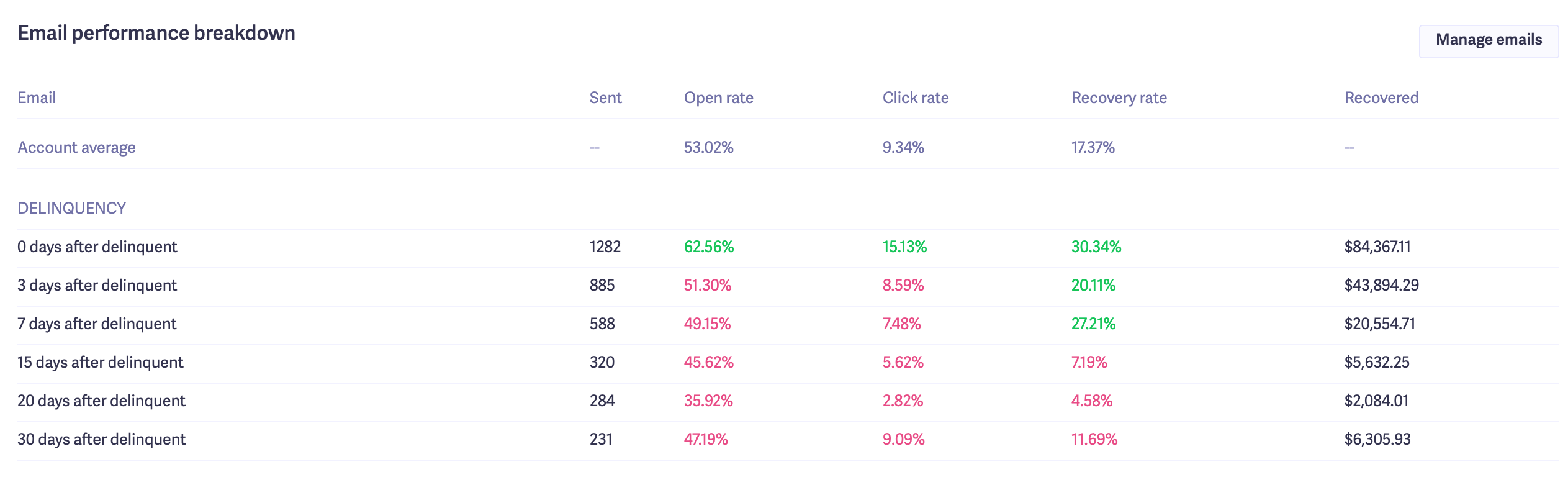The image, set against a stark white background, captures a small, detailed data table titled "Email Performance Breakdown." The table outlines various email performance metrics across several columns labeled from left to right: "Email Sent," "Open Rate," "Click Rate," "Recovery Rate," and "Recovered." 

The first row of the table represents the account average, displaying metrics such as a 53.02% open rate, a 9.34% click rate, and a 17.37% recovery rate. The specific numbers for "Emails Sent" and "Recovered" are not provided in this row.

Following the account average, the next section focuses on emails sent at different stages of delinquency. For emails sent on the same day as becoming delinquent ("0 days after delinquent"), 1,282 emails were dispatched, with a 62.56% open rate, 15.13% click rate, and 30.34% recovery rate, successfully recovering $84,367.11.

The final part of the data shows the performance for emails sent three days after becoming delinquent. For this period, 885 emails were sent, achieving an open rate of 51.3% and a click rate of 8.59%. The recovery rate and the amount recovered for this particular period are not disclosed in the given excerpt.